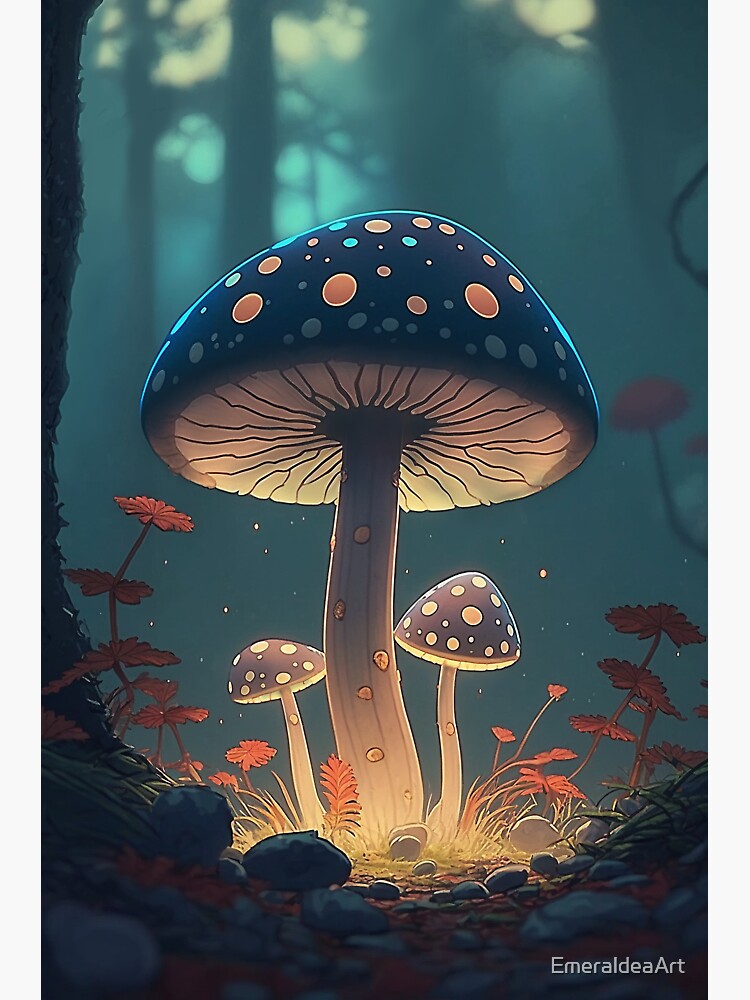In the dark, hazy forest backdrop of this digital illustration by Emeraldia Art, three distinct mushrooms take center stage. The largest mushroom, positioned centrally, features a dark blue cap adorned with orange and light blue polka dots of various sizes, and a brown stem detailed with subtle ridges. Below this prominent mushroom, two smaller versions mirror its design with shorter, slimmer stems and similarly patterned caps, albeit in lighter hues. A soft yellow glow emanates from beneath them, casting an enchanting light on the scene. The ground surrounding the mushrooms is dotted with dark blue-grey stones and vibrant orange plants with flowers and leaves. In the blurred background, tall trees with a dark green tint add to the dreamy, mystical atmosphere. The artwork is signed "Emeraldia Art" in white at the bottom right corner.